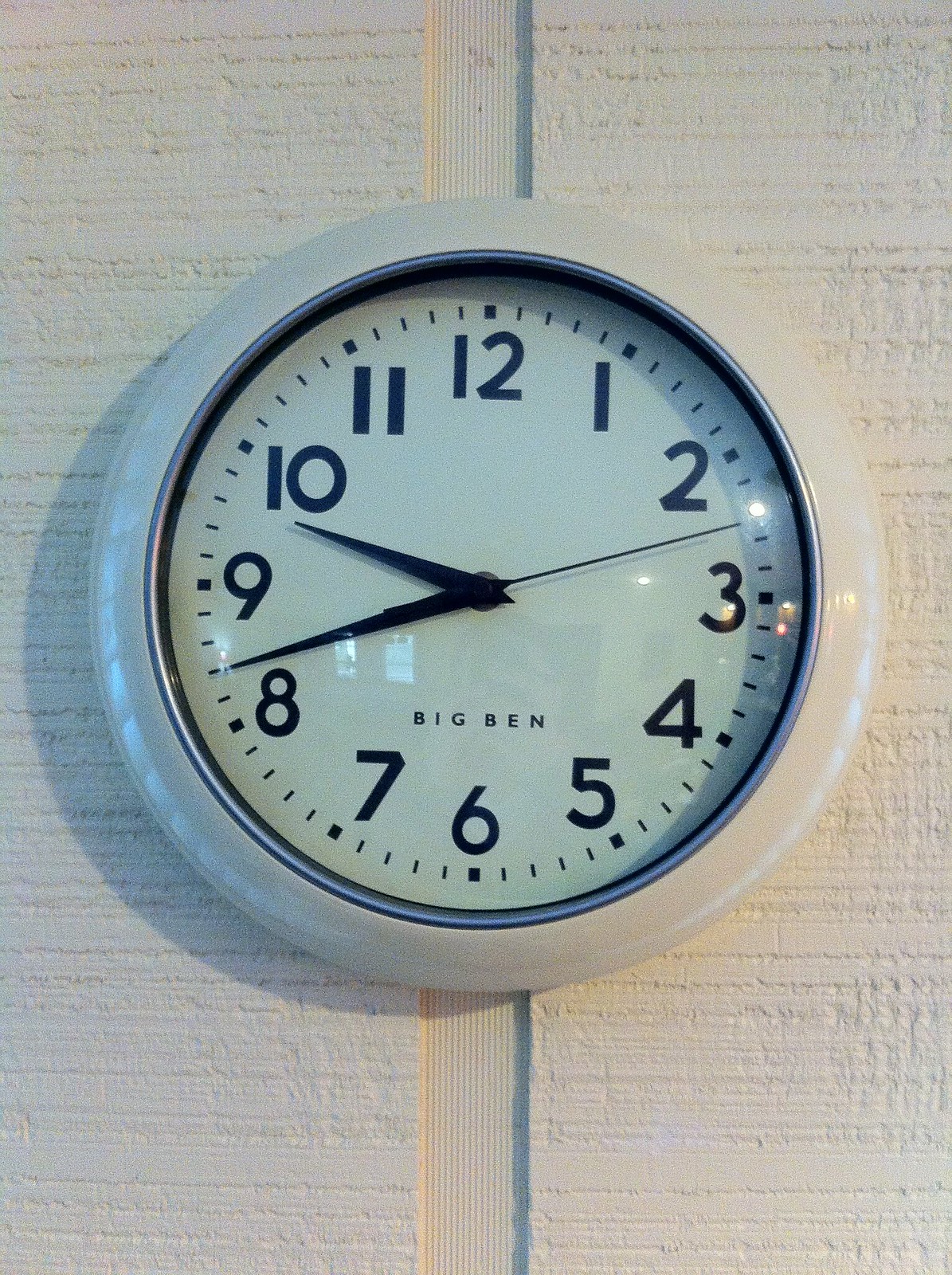The image features a wall with a pristine white stone surface, characterized by a pattern of vertical and horizontal lines. Against this backdrop is a clock with a sleek white body frame. The clock face is marked by bold dash marks at each hour, and it displays the numbers 1 through 12 in a clear, legible font. The hour hand is positioned between the 9 and 10 markers, while the minute hand is located between the 8 and 9 markers. Surrounding the clock is a big, elegant bed that adds to the room's aesthetic. There is also a glass object, possibly a window or a glass decoration, adding a touch of transparency to the scene.